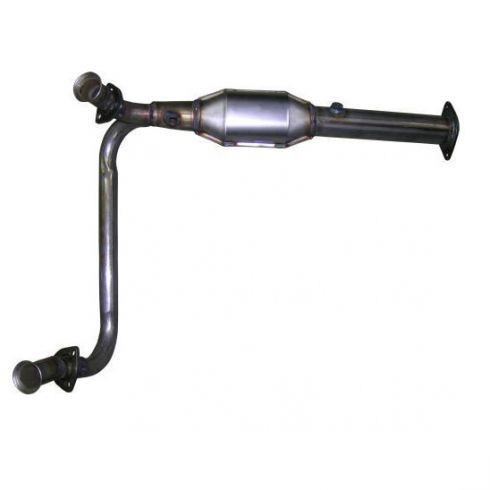The image showcases a mechanical device against a plain white background, emphasizing the object itself. The device appears to be a complex metal pipe assembly featuring an L-shaped configuration. The assembly includes a metallic black pipe that extends horizontally from the right to left, leading into a wider, silver-colored bulbous section at the center. This bulbous section splits into two narrower pipes; one extends to the top left and ends in a tubular spout, while the other bends downward on the left side and culminates in another similar spout. Additionally, there are bracket-like components on the ends of the pipes, suggesting points for potential connections or attachments. The precise function of the device is unclear, though its design hints at possible applications in plumbing or automotive systems.